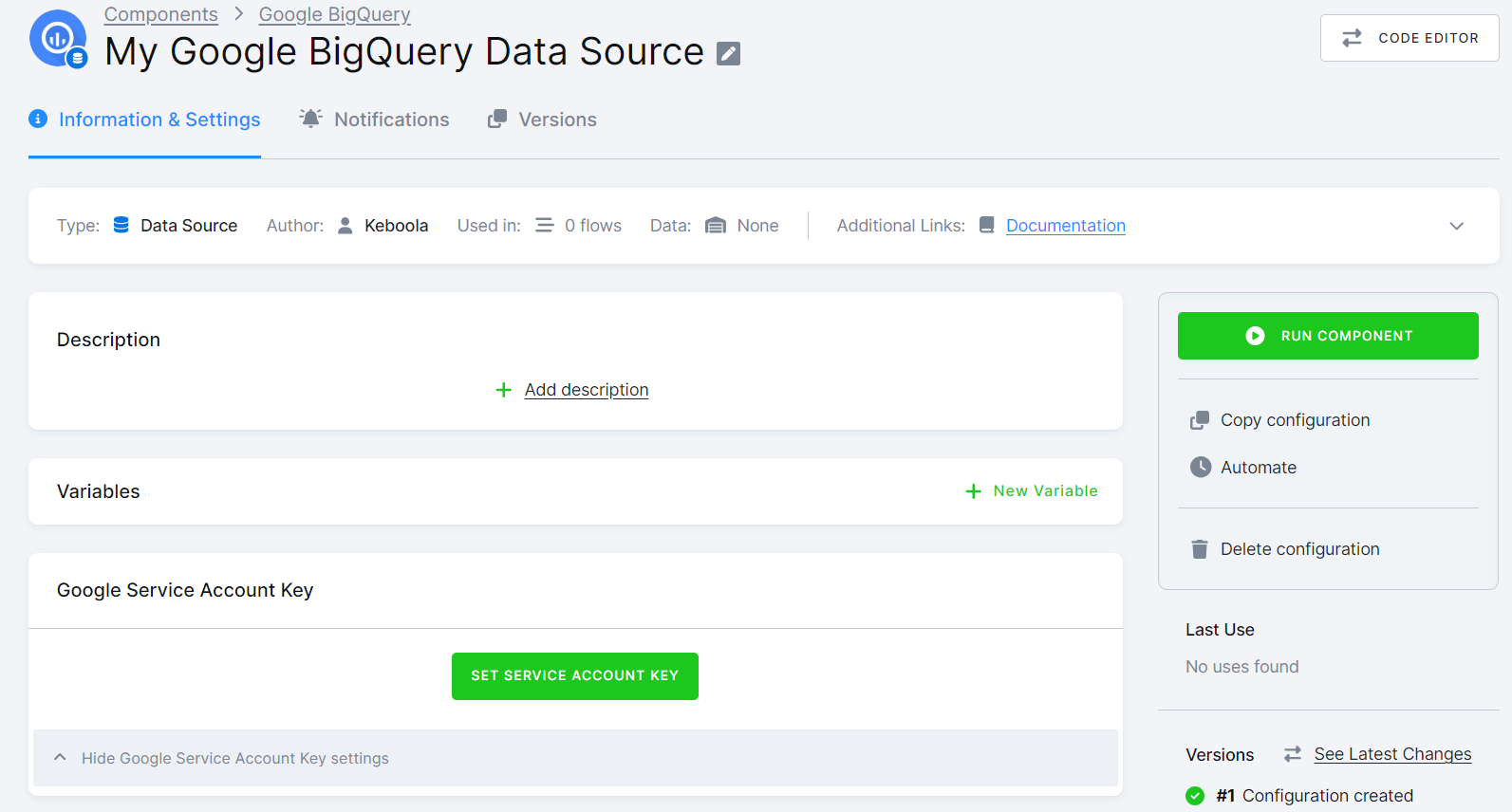This screenshot showcases a section of a website related to Google BigQuery. The background is primarily gray, with the top section featuring gray text that reads "components" followed by a forward arrow, and "Google BigQuery". Below that, in black font, it says "My Google BigQuery Data Source".

To the left, there is a blue circle with a white circle inside it. Below this circle, in blue font with a blue underline, indicating active selection, it says "Information", followed by "Settings". To the right, in gray font, it lists "Notifications" and "Versions".

In the main content area, there is a white rectangle containing descriptors in gray font: "Type", "Author", and "Used in", followed by blue text reading "Documentation". Under "Type", in black font, it states "Data Source". Under "Author", it lists "Keboola" in black font. Additionally, it indicates "Used in 0 Flows", followed by "Data: None" and "Additional Links". 

Below these details, there is another white rectangle titled "Description" in black font. Further down, another white rectangle is present, labeled "Variables".